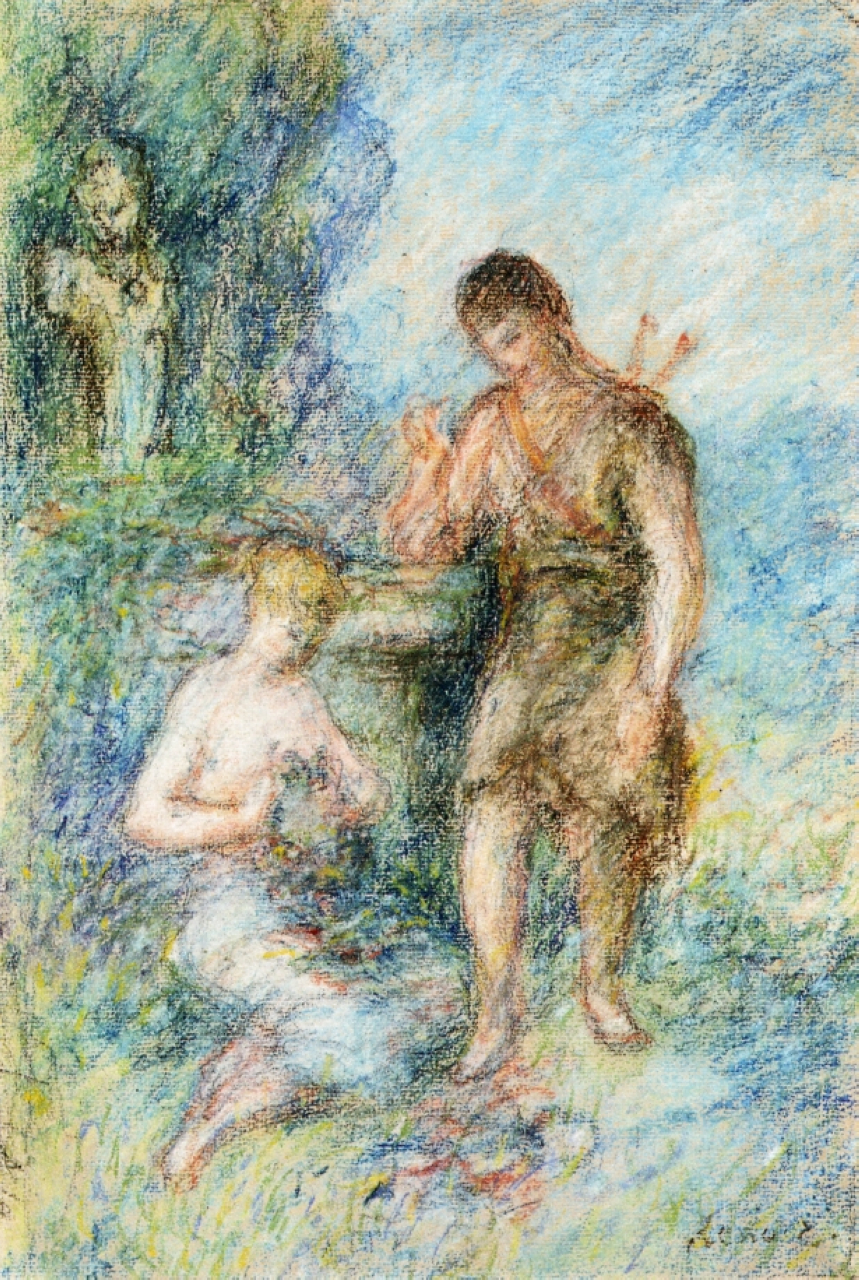This detailed painting, possibly a muted watercolor, appears to be of a scene reminiscent of ancient or medieval times. Centrally featured are two individuals: a young man standing and a young woman seated on the ground beside him. The man, adorned with arrows in a quiver strapped to his back, wears a minimalistic outfit akin to ancient attire. He looks down at the woman, smiling, as if engaging with her. The woman, with her blonde hair, seems to be holding something in her lap, though it's ambiguous whether it's flowers, a cat, or a dog due to the painting's soft and indistinct style.

The woman's attire is minimal, suggesting nudity. Surrounding them, the artwork features a variety of colors including white, blue, tan, brown, orange, black, lime green, gray, purple, and yellow, creating a serene, almost ethereal atmosphere. Behind and to the left is another figure, a bust wearing a medallion, looking downward. This figure is somewhat obscured but adds a layer of complexity and depth to the scene. The artist's signature is visible in the bottom right corner, indicating this painting, with its collection of soft, blended hues and intricate details, is likely a valued piece that one might expect to find adorning the wall of a refined household.